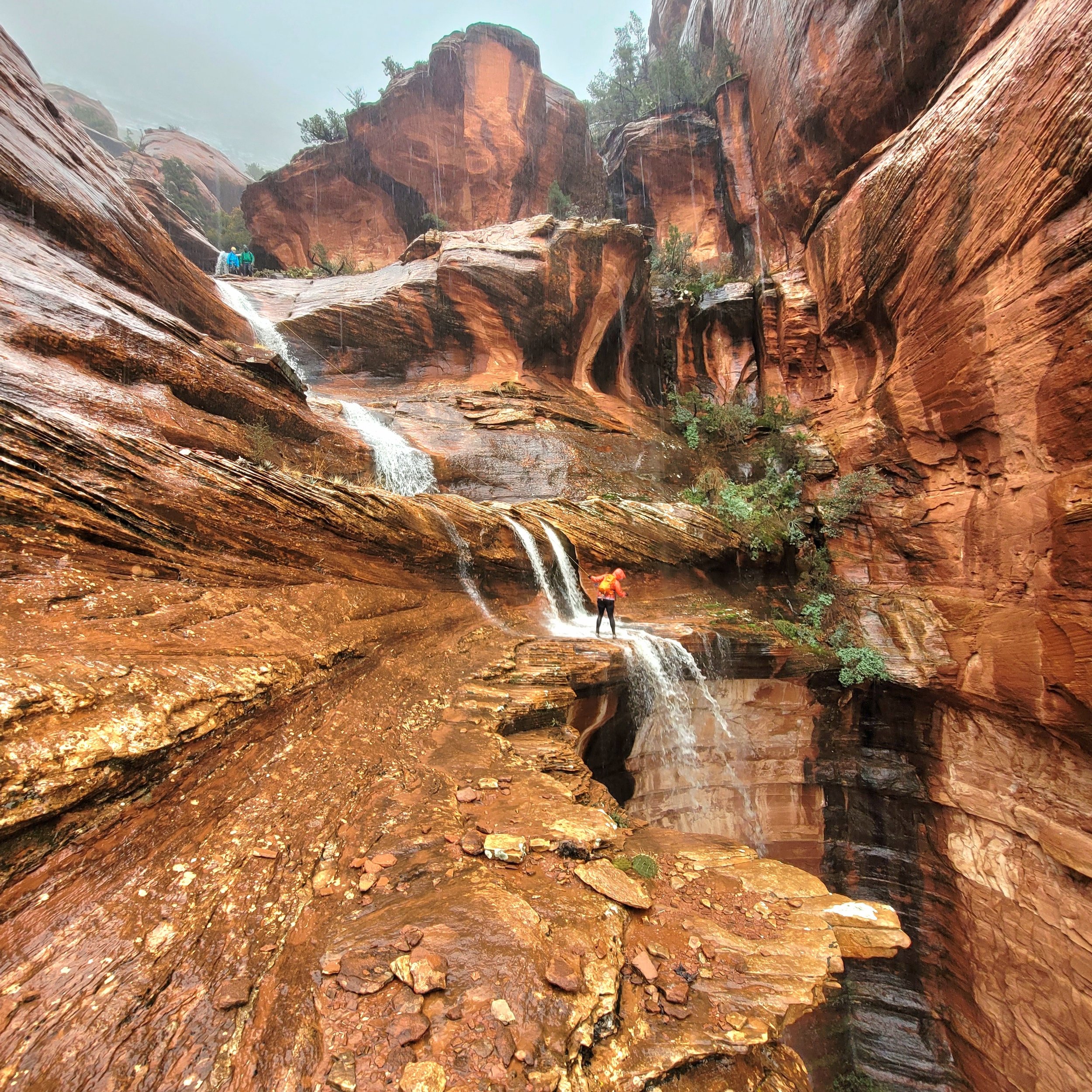The image depicts a multi-layered waterfall cascading over several ledges of rocks into a deep cavern below. At the top of the image, there is a mountainous background where the waterfall originates, with water flowing in from the top left. The rocks surrounding the waterfall range in colors from light and dark brown to orange and dark gray, exhibiting a rich, textured palette. Moss and greenery can be seen on some sections, particularly towards the right. The waterfall transitions through multiple tiers, not a single drop, giving it a layered appearance.

At the top of the waterfall, a couple of people can be seen standing, likely observing the scene below. In the middle of the image, a striking figure in an orange and black parka stands at the edge of the third level of the waterfall, surrounded by imposing rocks. The water here appears minimal as it continues its descent. Additionally, a woman dressed in similar attire is seen scaling down the wet, canyon-like walls, secured with ropes and hooks, while a few others watch from the top to ensure her safety. The entire scene is characterized by the rugged, eroded rock formations of reddish-brown color, accentuated by the elements over time. Trees and other vegetation grow sporadically within the rock, adding to the natural beauty of this expansive outdoor canyon.